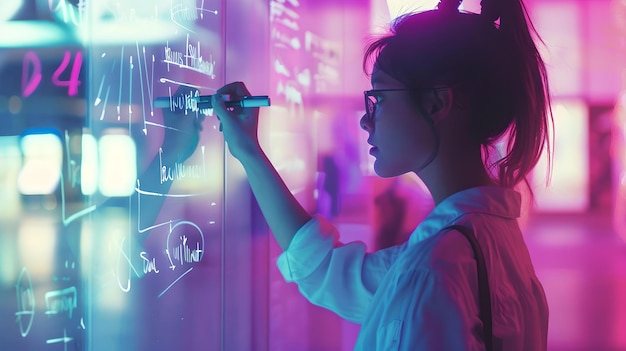In this vivid and moody photograph, an Asian woman is captured in profile as she writes on a futuristic whiteboard. She is positioned to the right of the image, wearing dark glasses and a collared, long-sleeved white blouse. Her hair is tied back in a ponytail, and her right arm is bent at the elbow, with her hand raised to a diagonal board covered in text and lines. The board, seemingly transparent and lit from behind, extends from the left side to the middle of the image, where she applies her marker or pen. The scene is set indoors, bathed in striking lighting: a pink glow envelopes her and reflects off her shirt, while a blue shine radiates from the left side. The illuminated colors—pink, purple, violet, and blue—create a cinematic and almost futuristic ambiance, highlighting the details of the woman's focused activity in writing numbers and figures on the board.